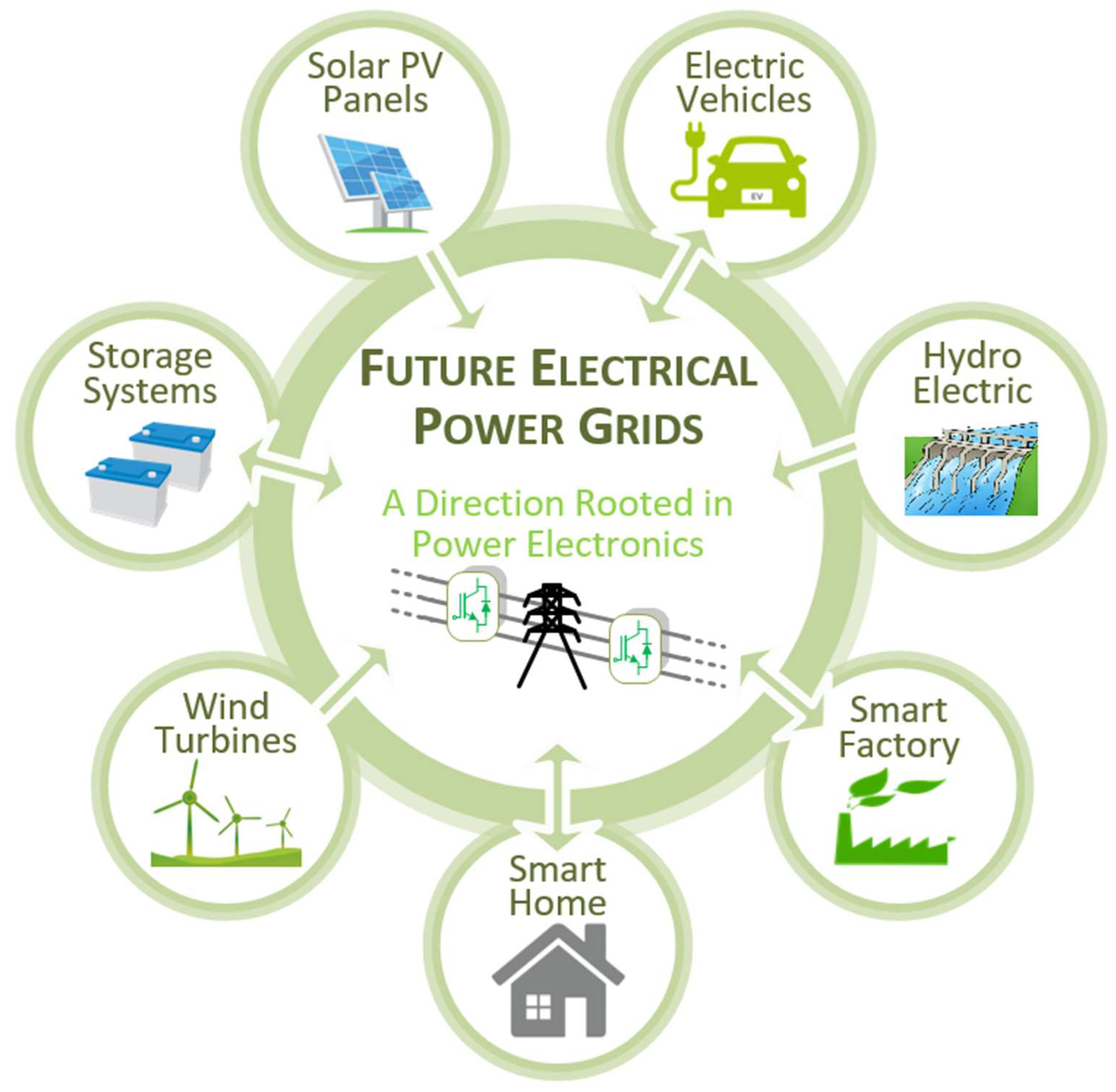This image is a detailed diagram illustrating the future of electrical power grids, emphasizing a direction rooted in power electronics. At the center is a large circle labeled "Future Electrical Power Grids: A Direction Rooted in Power Electronics," with a graphic of a transmission tower and lines beneath it. Surrounding the central circle are seven smaller circles, each connected by arrows and representing different components and destinations of the power grid.

Starting at the top left and moving clockwise:
1. **Solar PV Panels**: Depicted with a picture of solar panels, indicating the use of solar energy.
2. **Electrical Vehicles**: Shown with a car featuring a plug, highlighting electric vehicles as a key component.
3. **Hydroelectric Power**: Illustrated with a river, representing energy generated from water sources.
4. **Smart Factory**: Demonstrated with a factory chimney emitting green leaves, symbolizing eco-friendly manufacturing.
5. **Smart Home**: Illustrated with a house, showing the integration of smart homes in the grid.
6. **Wind Turbines**: Shown with three windmills, representing energy derived from wind.
7. **Storage Systems**: Depicted with two containers, suggesting energy storage solutions.

This comprehensive graphic provides a clear vision of how future electrical power grids will incorporate various renewable energy sources and distribute power efficiently to create a sustainable energy ecosystem.